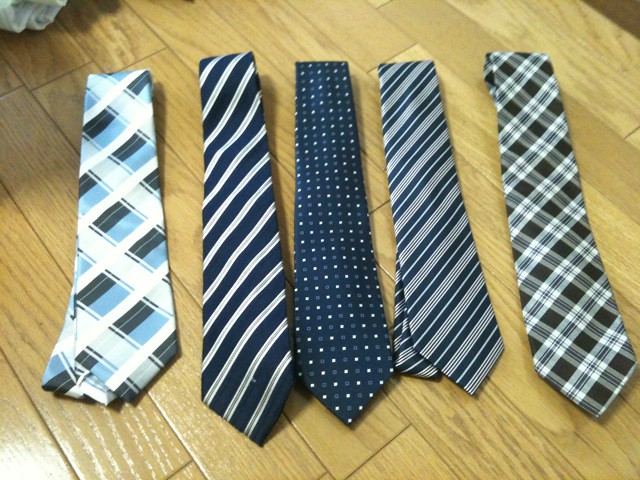An array of men's ties is displayed on a light blonde, narrow-board wooden floor. From left to right, the ties exhibit various intricate patterns, all featuring shades of blue prominently. The first tie on the left is light blue and dark blue with broad white stripes. Next is a predominantly blue tie adorned with diagonal thin white stripes and a slender silver stripe down the middle. The third tie showcases alternating small white and gray dots on a blue background. Following that is a tie designed with thick diagonal blue stripes interspersed with narrow gray stripes. Lastly, a gray and white crosshatch crochet pattern tie rounds out the collection. The detailed and varied designs of these ties create a visually appealing assortment.